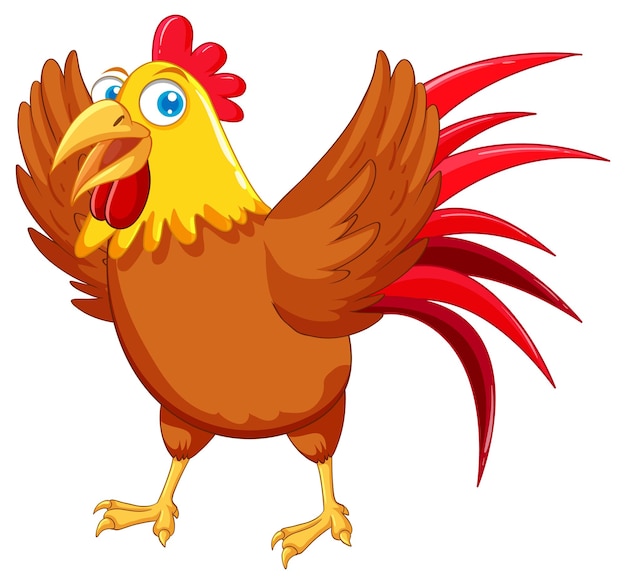The image is a colored cartoon drawing of a joyful, humanized rooster. Shown in a three-quarter view with its face turned to the left, the rooster is animatedly walking on its hind legs with wings spread out as if celebrating. Its body is mostly light brown, complemented by bright yellow head and neck, and mustard-colored beak that is open mid-expression. The rooster's eyes are large, cartoonish, and blue, adding to its friendly demeanor. It has a prominent red comb and wattle, and its vibrant red tail feathers fan out to the right, partly covered by its wings making the connection point unclear. The legs and claws are tan. The entire rendering is set against a plain white background, emphasizing the rooster's exuberant and lively character. The illustration, outlined and filled with color, exudes a cheerful and approachable vibe, reminiscent of a sports mascot or animation character.